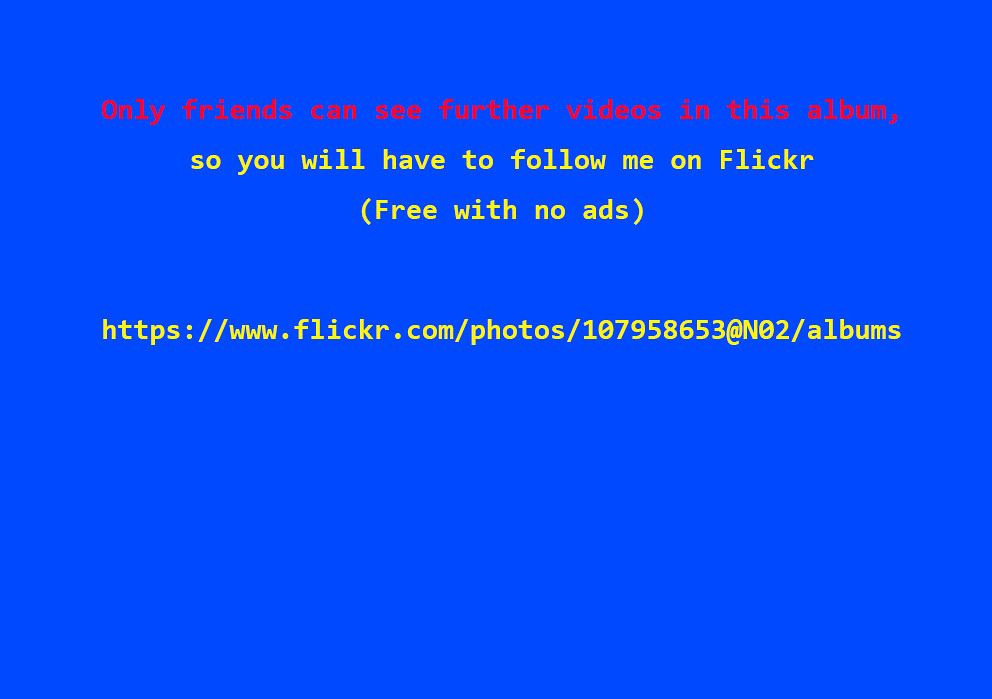The image depicts a widescreen monitor with a medium blue background. Displayed on the screen is a sequence of text lines in bright red and yellow. At the top, written in red text, it says, "Only friends can see further videos in this album." Directly below, in yellow text, the message reads, "so you will have to follow me on Flickr." Continuing in yellow, the next line within parentheses states, "(free with no ads)." Following a line break, another line in yellow text shows the URL: "https://www.flickr.com/photos/107958653@N02/albums." The bottom half of the image remains blank, simply extending the blue background without any additional text or elements.